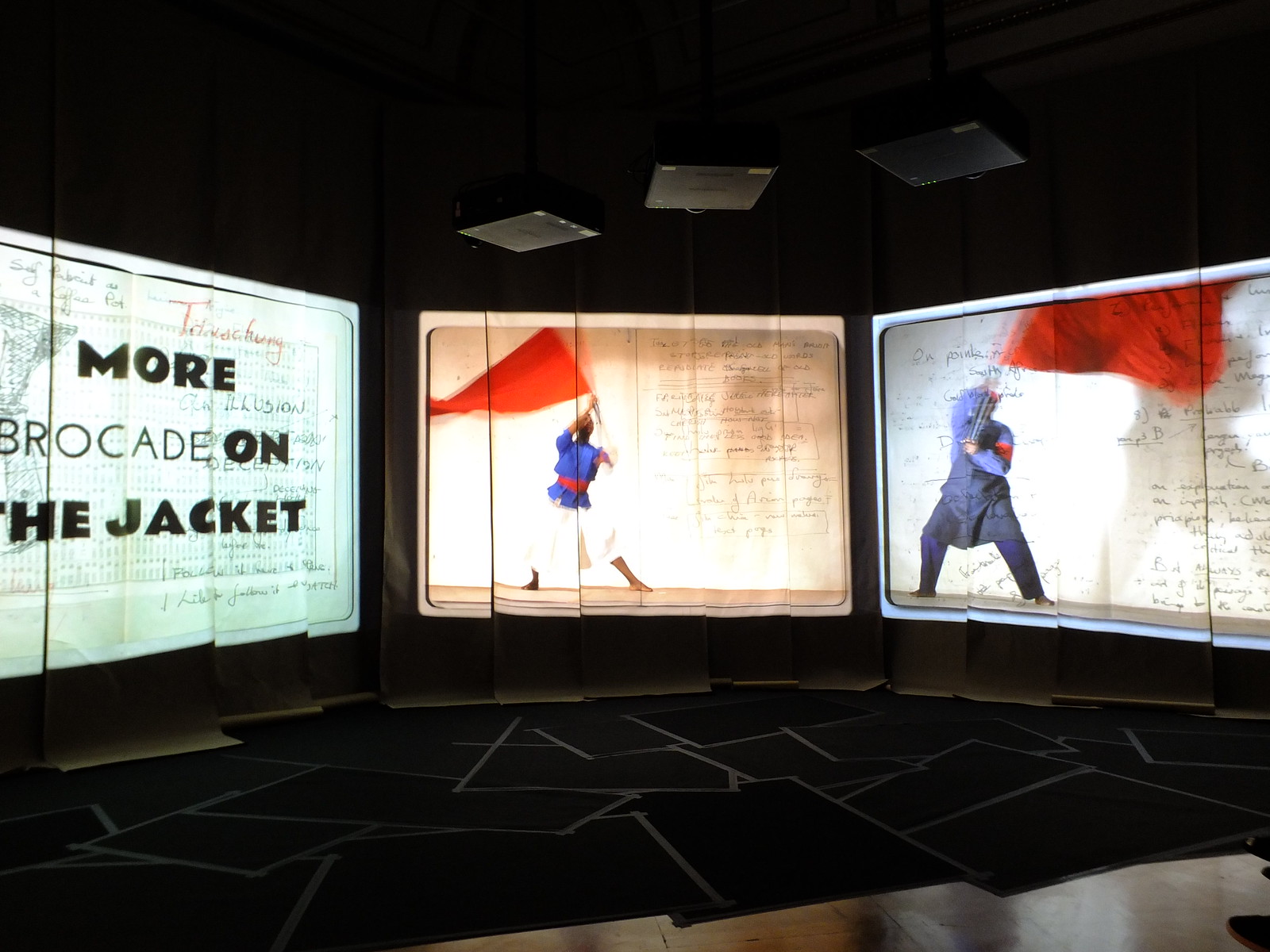This photo depicts a darkened, possibly museum-like environment, illuminated by three prominently displayed screens arranged left to right. The left screen is partially cut off but clearly shows bold black text stating "War" and "Jacket" amidst other partially obscured words. The middle screen features a person of color in a blue shirt, white baggy pants, and a red belt, holding a large red flag aloft while barefoot and looking up. The right screen displays a light-skinned individual dressed in a dark blue shirt and pants, also waving a large red flag. Both individuals are positioned against a backdrop filled with text and papers. Above the screens, three ceiling lights cast a glow, while below lies a jumble of black rugs or wood, contributing to the intricate, staged setting.